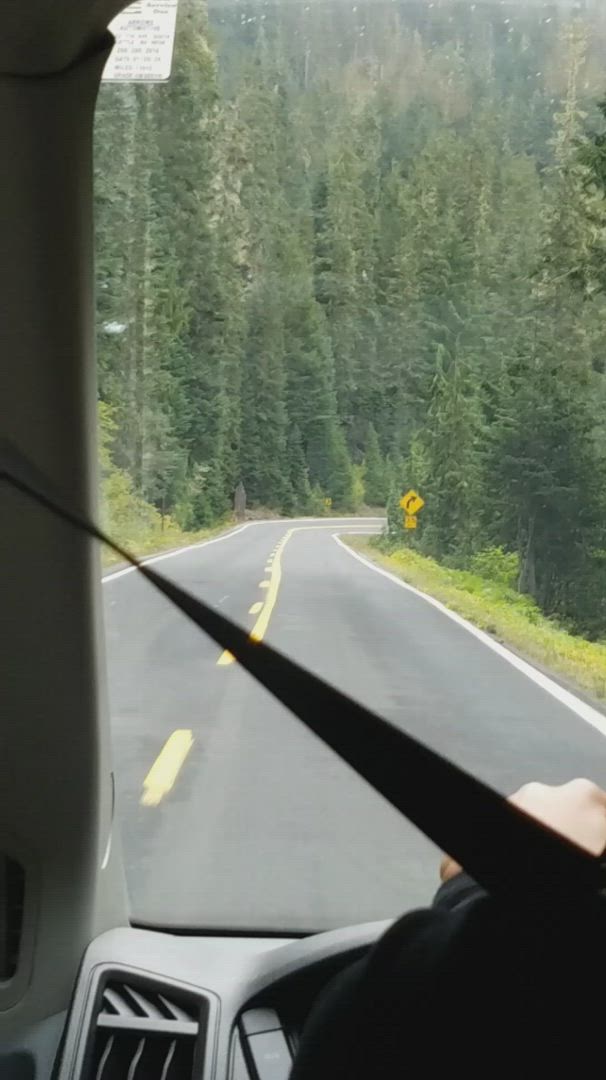The photograph captures a driver's-eye view navigating a winding mountain road during a clear day. The scene reveals a well-maintained, paved road marked by a central yellow dashed line, which transitions into a dashed-slash-solid line as it approaches a downhill right turn. Prominently displayed in the center of the shot is a yellow right-turn indicator sign, guiding the driver through the mountainous terrain.

Tall trees densely line both sides of the road, casting shadows that contrast with the bright daylight. The road edges are clearly delineated by white boundary lines. In the bottom right corner of the image, part of the driver’s white arm, clad in a black sweater, grips the steering wheel, providing a sense of real-time navigation. The car's gray dashboard and a black seatbelt cutting diagonally across the frame add context to the interior setting. On the left side of the image, the edge of the car's windshield pillar frames the scene, emphasizing the enclosed yet expansive view ahead as the road curves right and descends into the lush greenery of the mountain landscape.